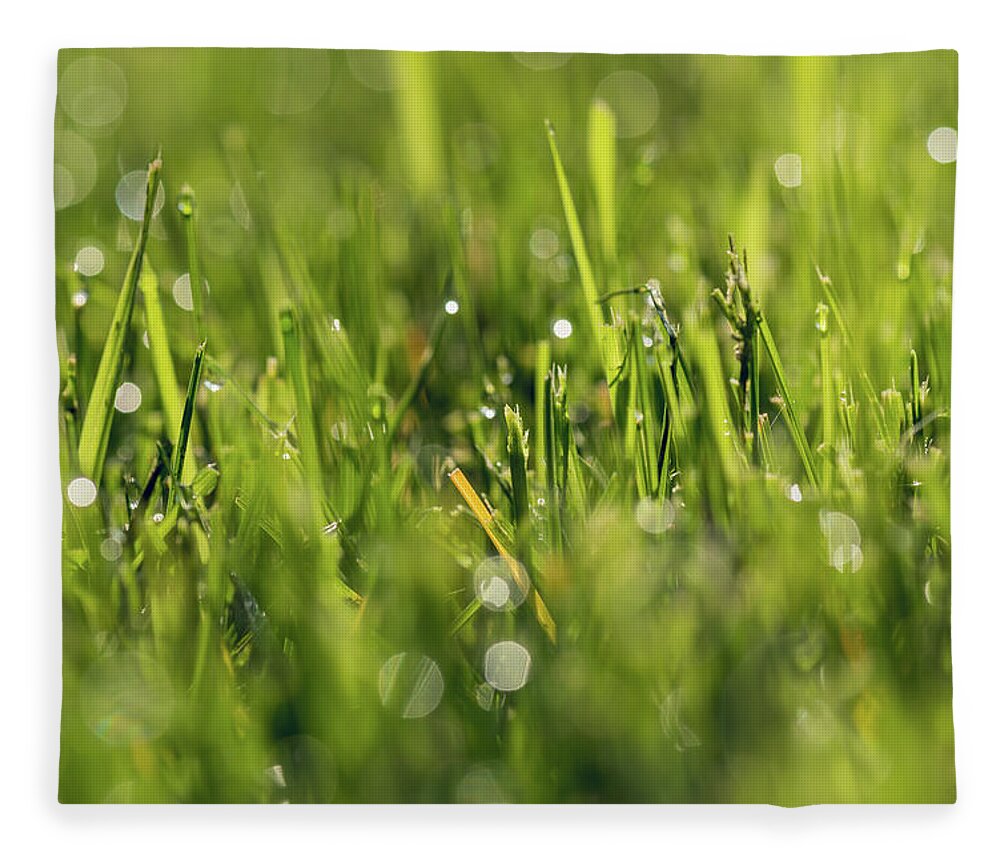The image is a close-up shot of grass at ground level, predominantly showcasing green blades with a few taller and shorter ones mixed together. In the middle of the frame, the grass is sharply in focus, while the foreground and background are blurred. The photograph captures droplets of water, likely from rain or dew, dotting the blades and creating reflective patterns. A couple of brown grass blades are visible towards the center, adding contrast to the lush green. The edges of the image are uneven, giving it a dynamic feel. A hint of morning light adds a soft glow, and there are some tiny weeds and possibly a few black sticks interspersed amongst the grass. Some water droplets on the camera lens add to the overall wet, fresh, and slightly misty ambiance.